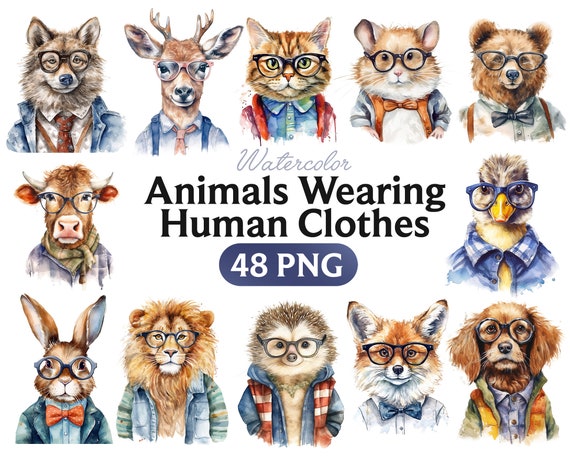In this detailed illustration with a white background, a diverse array of animals are artfully depicted in watercolor, dressed in a variety of human clothing and accessories. The animals, which include a wolf, deer, cat, mouse, bear, cow, rabbit, lion, porcupine, fox, dog, and duck, are positioned around the border of the image, creating a lively and whimsical frame. Each animal is adorned with glasses, emphasizing a scholarly demeanor, and dressed in an assortment of outfits, including bow ties, suspenders, cardigans, and different types of shirts in shades of blue, red, and occasional pops of orange. The top edge features five animals, the sides each have three, and the bottom edge has another five, completing the rectangular border. At the center of the image, the text "watercolor, animals wearing human clothes, 48 PNG" is prominently displayed, indicating that this might be an artistic set available for purchase, potentially teaching step-by-step watercolor techniques. The styling and details unify the illustrations, presenting a charming and cohesive collection of anthropomorphized animals.